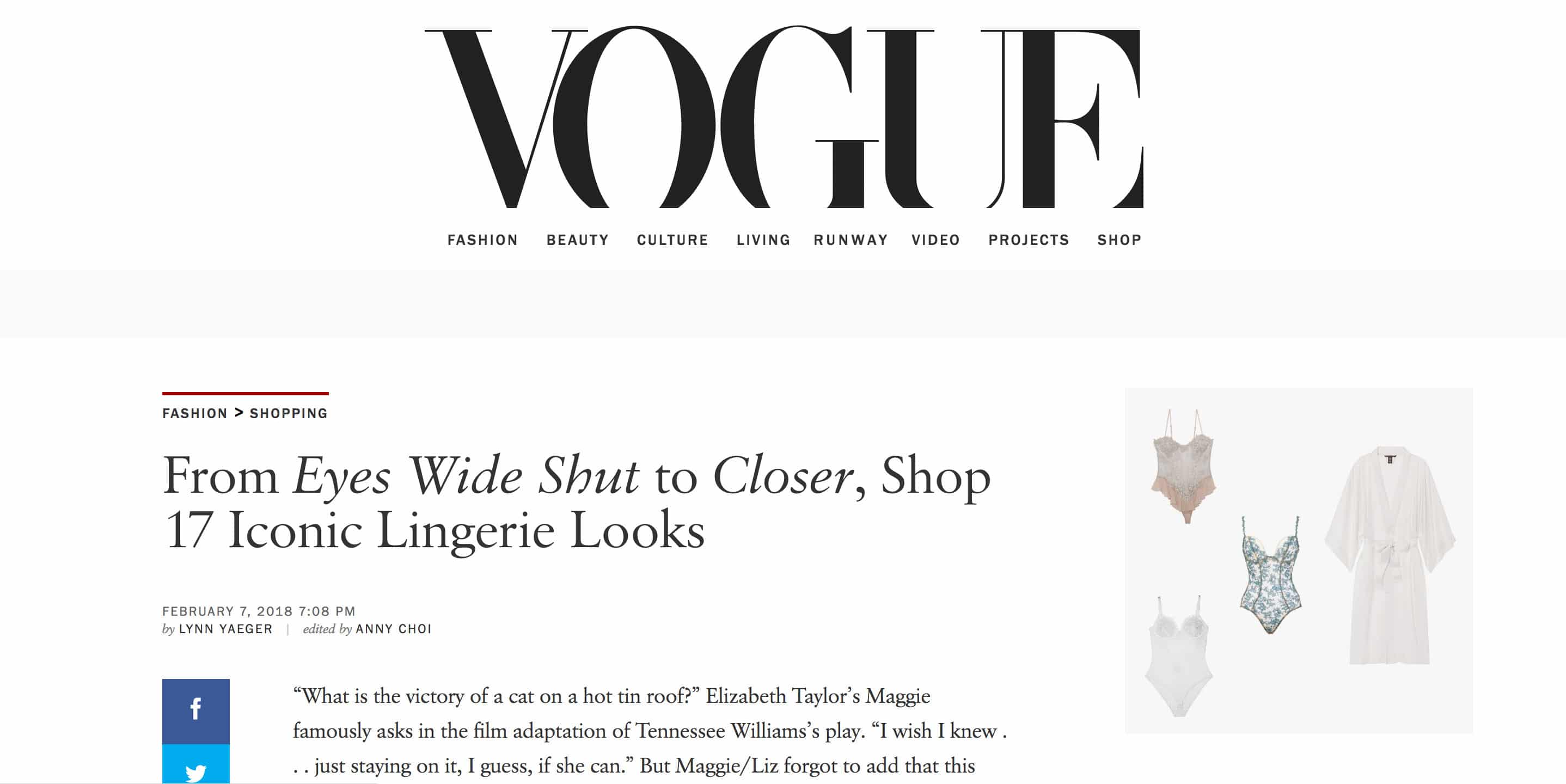At the top of the page, the word "Vogue" is prominently displayed in large, bold, black letters. Just below, a navigation menu lists categories: Fashion, Beauty, Culture, Living, Runway, Video, Projects, and Shop. Underneath this menu, a thin red line separates it from the next section, which reads "Fashion and Shopping." 

Further down, the title "From Eyes Wide Shut to Closer: Shop 17 Iconic Lingerie Looks" is positioned, followed by the date and time: "February 7th, 2018, 7:08 PM" and the author credit "by Lynn Yeager" and "edited by Annie Choi." Below these details, two social media icons are displayed: a blue box with the letter 'F' for Facebook and another blue box with a bird silhouette for Twitter.

On the right side, within quotation marks, there's a notable quote: "What is the victory of a cat on a hot tin roof?" Elizabeth Taylor’s Maggie famously asks in the film adaptation of Tennessee Williams' play. The quote continues, "I wish I knew. Just staying on it, I guess. If she can..." but oddly, the quote trails off, adding an element of intrigue.